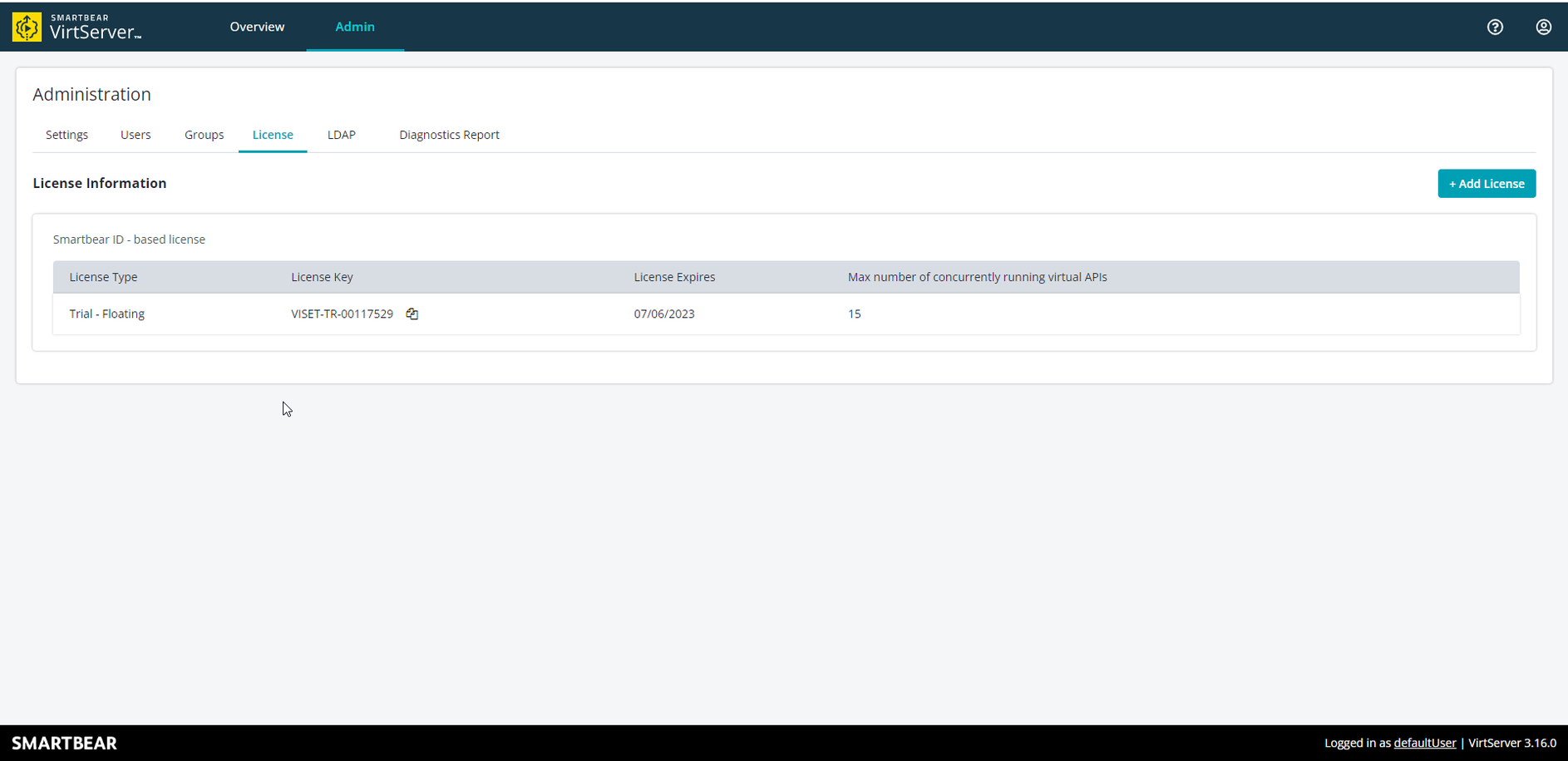In the top left corner of the image, there is white text that reads "SmartBean Virch Server." Adjacent to this text on the right is a yellow icon featuring a black arrow pointing upwards and to the right. This icon is situated within a blue area. Further to the right, the words "Overview" and "Admin" are displayed, with "Admin" being underlined and colored in blue. On the top right corner of the image, a question mark icon is visible next to an icon resembling a person.

Directly below this, there is a white chart titled "Administration." The chart lists several items including "Settings," "Users," "Groups," "License," "LDAP," and "Diagnostics Report." Beneath this section, in black text, it reads "License Information." To the right of this heading, a blue button labeled "Add a License" is present.

Further down, the text "SmartBear ID Based License" appears above a gray chart. This chart details various license-related information under the columns "License Type," "License Key," "License Expires," and "Max Number of Concurrently Running Virtual APIs." The specific details listed are:
- License Type: Trial Floating VSET
- License Key: TR 0011 7529
- License Expires: 07/06/2023
- Max Number of Concurrently Running Virtual APIs: 15